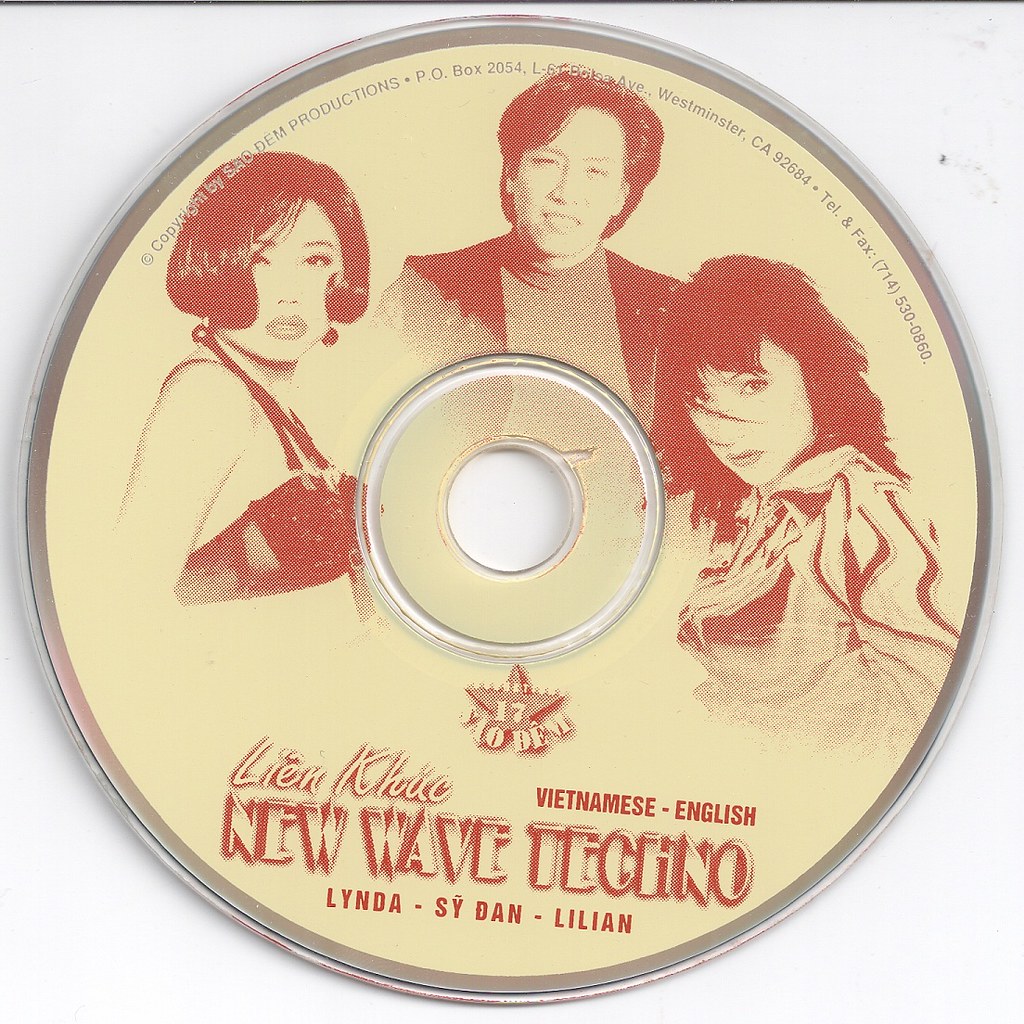The image features a close-up of a CD disc with a beige background and a grayish border. The disc's central hole is surrounded by intricate drawings in a reddish-black hue, giving it an old, vintage appearance. The artwork highlights three individuals: a man and two women, arranged around the disc. 

The central figure is a man wearing a black vest over a lighter-colored undershirt. On his left (the viewer’s right), there is a woman with short black hair and a small bikini top with straps over her shoulders. She has her body turned to the right but is looking forward. On the man’s right (the viewer’s left), there is another woman with shoulder-length black hair wearing a flowy jacket and a lighter-colored garment, featuring some red stripes. She is looking directly at the viewer with her head slightly turned to the left.

At the top of the CD, the text describes the production details, with an upper-right section indicating "Vietnamese/English." At the bottom, a cursive script reads "Lien Kyke," followed by the genre "New Wave Techno." Below this, the names "Linda, Sai Dan, and Lillian" are listed, along with a star logo featuring the number 17.